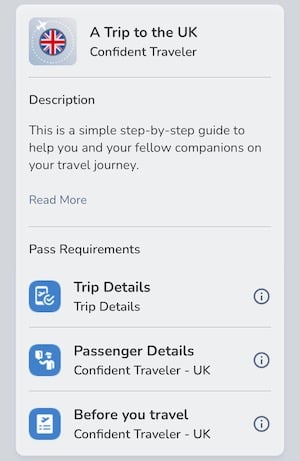Here is a cleaned-up, detailed caption for the image described:

---

**Image Description:**

The image showcases a minimalistic web page displayed on a cell phone screen, devoid of any cell phone icons, focusing solely on the webpage content. The main view is a gray square box, and centrally positioned within it is a smaller, lighter gray box. 

At the top of this inner box is an icon featuring a British flag with a small airplane circling around it, symbolizing travel. Next to the icon, the text reads "A trip to the UK, confident traveler" in black. Directly below this heading is a gray bar that introduces a section labeled "Description," which provides a brief explanation: "This is a simple step-by-step guide to help you and your fellow companions on your travel journey."

Following this is a hyperlink styled in a bluish-gray color labeled "Read more." Below, another gray bar introduces the "Pass Requirements" section. This section contains a blue box with an icon and text that reads "Trip details," alongside another icon on the right for further information.

The next segment is titled "Passenger details, confident traveler, UK," featuring another blue box with an icon on the left and an additional information icon on the right. At the bottom of the inner gray box, a final blue box is labeled "Before you travel, confident traveler, UK," also accompanied by an information icon on the right, represented as a small circle with an 'i' inside it.

---

This caption maintains the detailed description of the webpage elements as specified.